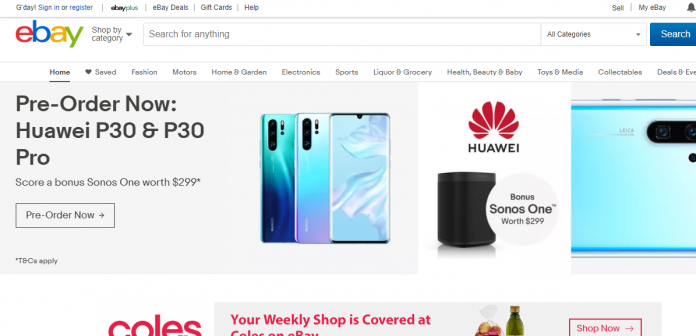The top part of the page features a white and black header that reads, "Gee, battery day, so maybe good day." Below this, "Sign in" is displayed in blue, followed by "Register" in black. A thin gray vertical line separates different sections.

Immediately to the right, a black text reads "eBay," followed by a green "plus" icon. Another gray vertical line separates this from "eBay deals," "gift cards," and "help".

Further to the right, another section begins with "Sell" in black text, followed by a thin gray vertical line. Next, "My eBay" appears alongside a gray bell icon.

Beneath the header, the eBay logo is prominently displayed, with the 'E' in red, 'B' in blue, 'A' in yellow, and 'Y' in green. Adjacent to the logo, in black text, "Shop by category" is followed by a list of categories:
- Home (highlighted with an underline and a heart icon)
- Fashion
- Motors
- Home and Garden
- Electronics
- Sports
- Liquor and grocery
- Health and beauty
- Baby
- Toys and media collectables
- Deals
- E, V, E (cuts off here)

The subsequent section has a gray background with "Pre-order now..." written in black, promoting the "HUAWEI P30 and P30 Pro." It mentions a bonus Sonos worth $299. Below, there is a black-outlined button labeled "Pre-order now." An image of three phones is displayed, presumably the HUAWEI P30 and P30 Pro models.